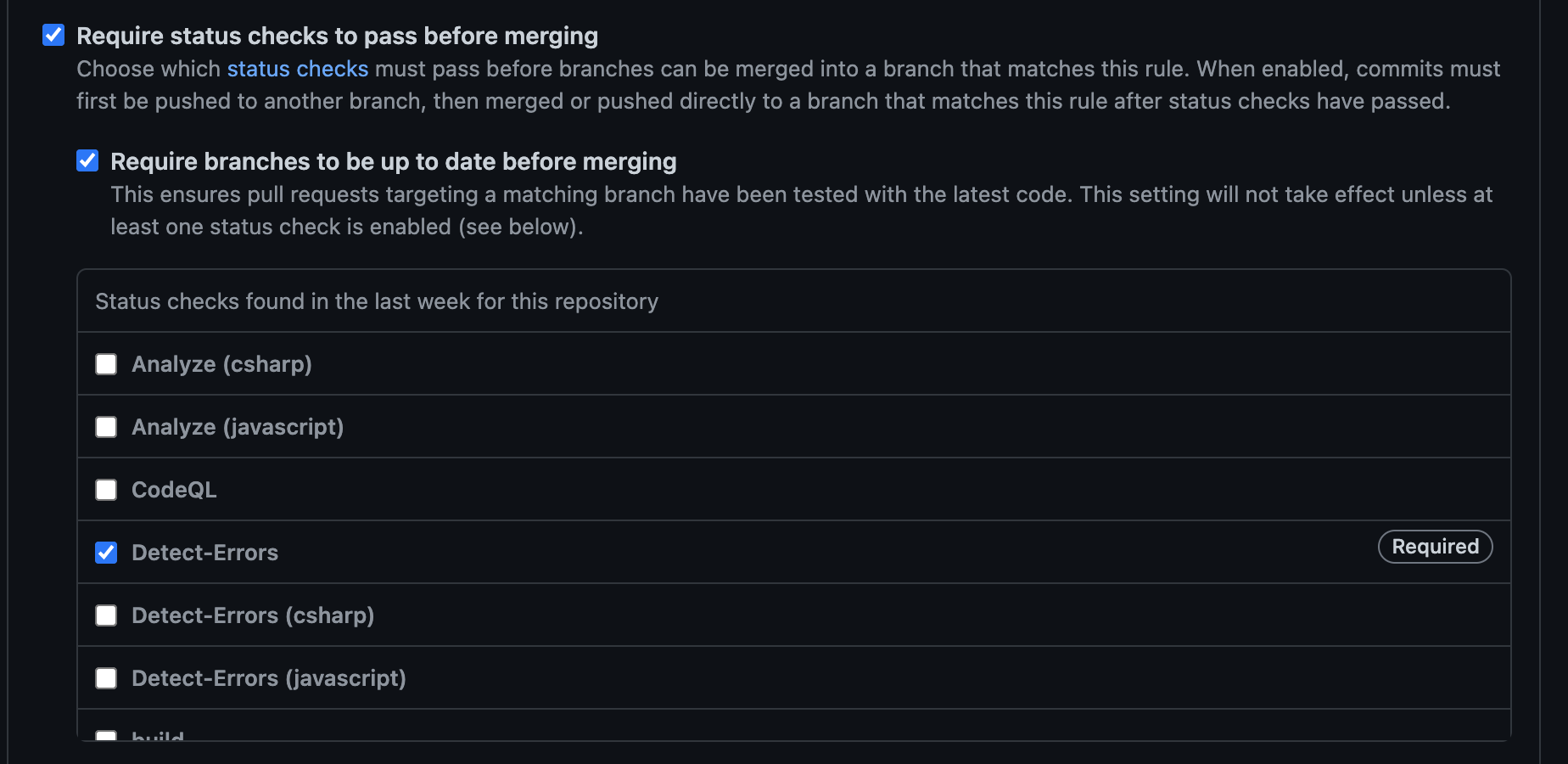**Detailed Caption:**

The image depicts a technical webpage interface related to programming, specifically focusing on merge settings for code repositories. At the top of the page, there is a checkbox labeled "Require status checks to pass before merging," which is checked. Below this, a detailed description explains that users must choose which status checks must pass before any branches can be merged into a branch that adheres to this rule. It is further articulated that any commits that are not enabled must first be pushed to another branch and then merged or directly pushed to a branch adhering to this rule, only after the status checks have successfully passed.

Another checkbox labeled "Require branches to be up to date before merging" is also checked, indicating that branches must be current before they can be merged. Below these checkboxes, there is a table listing the "Status checks found in the last week for this repository." The status checks include:
- Analyze C#
- Analyze JavaScript 
- CodeQL
- Detect errors (listed multiple times for different languages)
  - Detect errors: C#
  - Detect errors: JavaScript

Among these status checks, only the "Detect errors" checks are actively required, as indicated by the corresponding checkboxes and the word "required" to their right. 

The background of the interface is black, with white text, providing high contrast for readability.